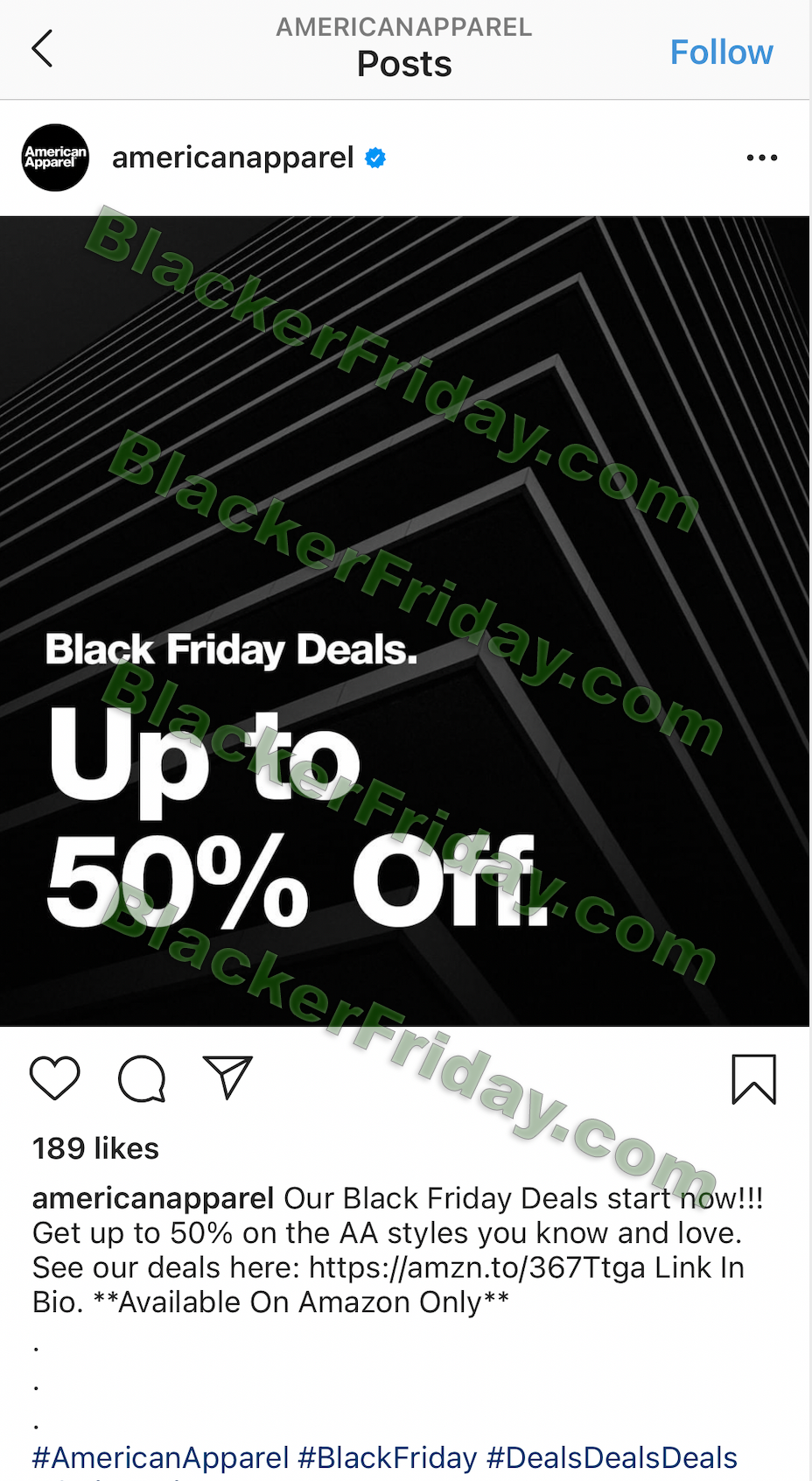This screenshot depicts an Instagram post by the user "American Appel" showcasing a Black Friday sale advertisement. At the top left corner, the username and timestamp of the post are visible. The central portion of the screenshot features the advertisement, highlighting "Black Friday deals up to 50% off" in bold, white text against a black square background. The square contains a subtle triangle-like design pattern. Overlaid on the image are four green watermarks reading "BlackerFriday.com," arranged diagonally from the bottom left to the top right corner. Below the advertisement, the caption reads: "Our Black Friday deals start now. Get up to 50% off the AA styles you know and love." The post has garnered 189 likes.